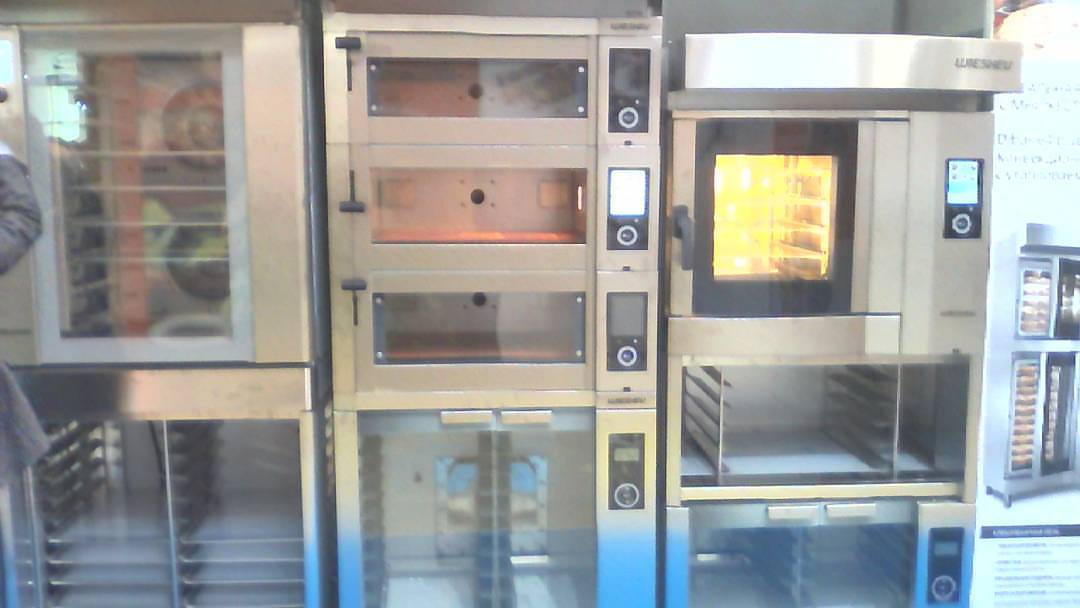This image is of a wall inside a commercial bakery, featuring an array of stacked, stainless steel appliances that resemble microwaves and ovens. The appliances are aligned in rows and columns, creating a sleek, industrial appearance. Starting from the left, the topmost appliance has a single glass door that allows visibility straight through, showing multiple shelves inside. Below it is another appliance with two rows of shelves, designed for baking items on sheets.

In the middle section, three smaller, black appliances with circular buttons that look almost like iPods are stacked on top. Below these, there's a larger stainless steel appliance that appears to be a proofer with spinning racks typically used for proofing bread. This proofer has a clear glass front, as do all the appliances, allowing a view of empty racks inside.

To the right, the top appliance features an illuminated interior, and below it is a small shelved section. Further down, there is another shelved oven, contributing to the uniform, functional look. Each appliance has digital displays and control panels for setting time and operation modes. Overall, the image captures the clean, efficient layout typical of a busy, well-equipped bakery or commercial kitchen.